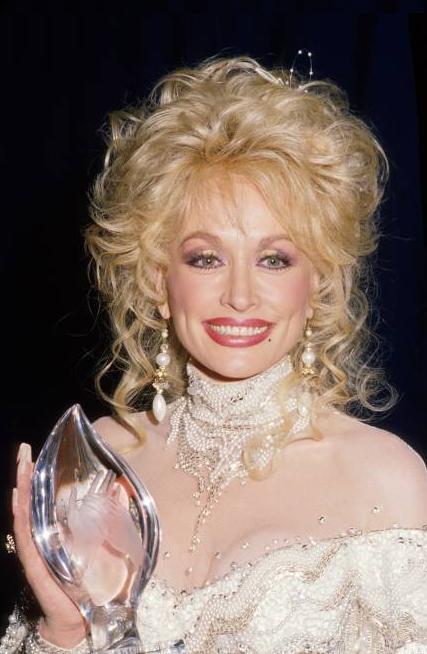This photograph features Dolly Parton against a stark black background, giving the impression she is floating in a dark void. Dolly is captured from the chest upwards, adorned in a high-collar, sheer white sequin dress. The dress showcases sequins and beads around her neck and mid-chest, with a sheer section from her upper chest to her neckline. She accessorizes with dangling gold and pearl earrings and a substantial gold ring on her ring finger. Dolly clutches a teardrop-shaped, see-through glass trophy in both hands, featuring two hands holding each other in a design. 

Her wavy, medium-length blonde hair cascades around her head, framing her face which is enhanced with dark mascara and vibrant red lipstick. The distinctive beauty mark on her face further accentuates her makeup. She wears a radiant smile, exuding her signature charm and elegance. The trophy, resembling a flame or swirl and fitting snugly within her grasp, adds a celebratory element to this striking image of the renowned country singer.